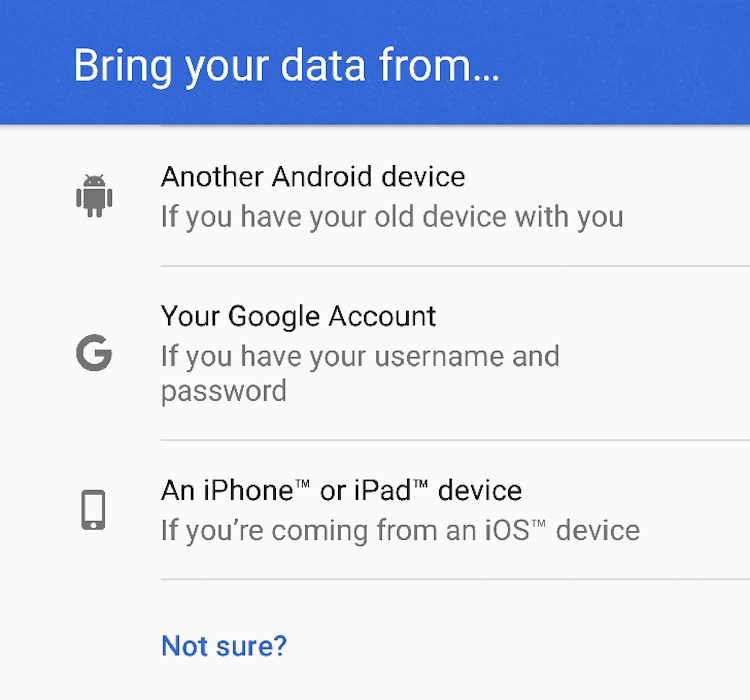In the image, there is a screen divided into several sections, each providing instructions for transferring data from different devices. At the top of the screen, there is a header with white text on a blue background that reads, "Bring your data from...". 

Below this header, there are instructions for transferring data from another Android device. To the left of this message, there is an icon of a robot. Beneath this text, there is a light gray horizontal line.

Further down, the next section starts with a large capital "G" on the left side. Next to it, the text reads, "Your Google account". Below this, the instructions mention that you will need your username and password. Another light gray horizontal line separates this section from the next.

At the bottom, there is a section indicating options for data transfer from an iPhone™ or iPad™. This section features an icon of a cell phone. The text next to the icon says, "If you’re coming from an iOS™ device". 

At the very bottom, in blue text, there is a question marked "Not sure?" The background of the entire screen is a light gray color, providing a clear and organized layout for the user to follow.